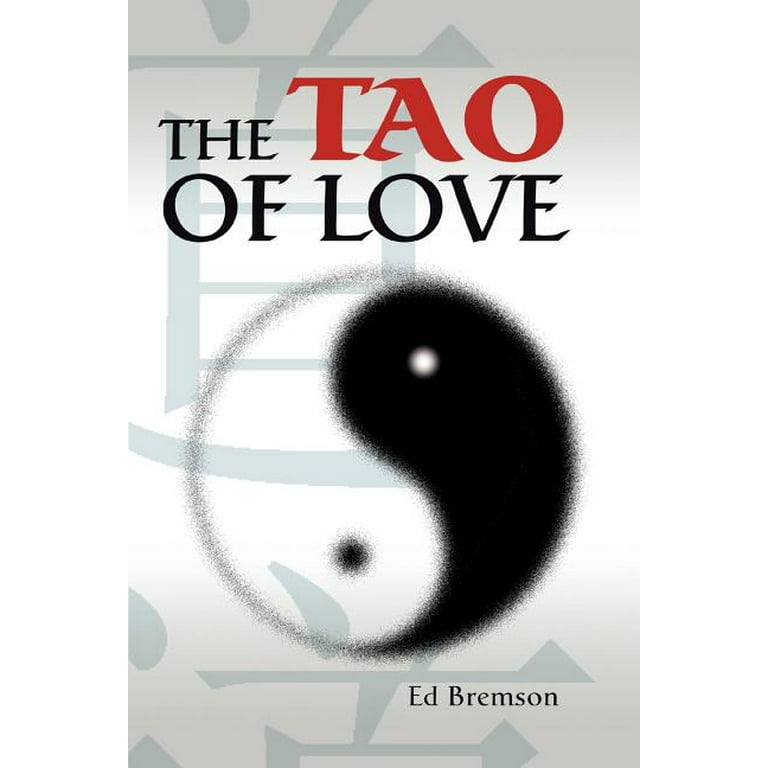The image is a detailed cover of a book titled "The Tao of Love" by Ed Bremsen. Central to the cover is a prominent black and white yin-yang symbol, appearing as if it were spray-painted with a perfect gray circle containing the harmonious interlocking black and white shapes. The word "Tao," spelled T-A-O, stands out in large, red brush-stroke letters, while the rest of the title, "of Love," is written in stark black font below it. The author's name, Ed Bremsen, is placed in the bottom right corner. Behind the central text and yin-yang symbol lies a subtle background of grayish Asian characters, adding an extra layer of depth without overshadowing the main elements. The overall color scheme of the cover consists of shades of gray, black, and white, maintaining a cohesive and tranquil visual theme, while the red "Tao" provides a striking contrast. This meticulously designed cover has a tall, rectangular shape, much like a traditional book, and appears to be a digital illustration, hinting at it potentially being an e-book cover.